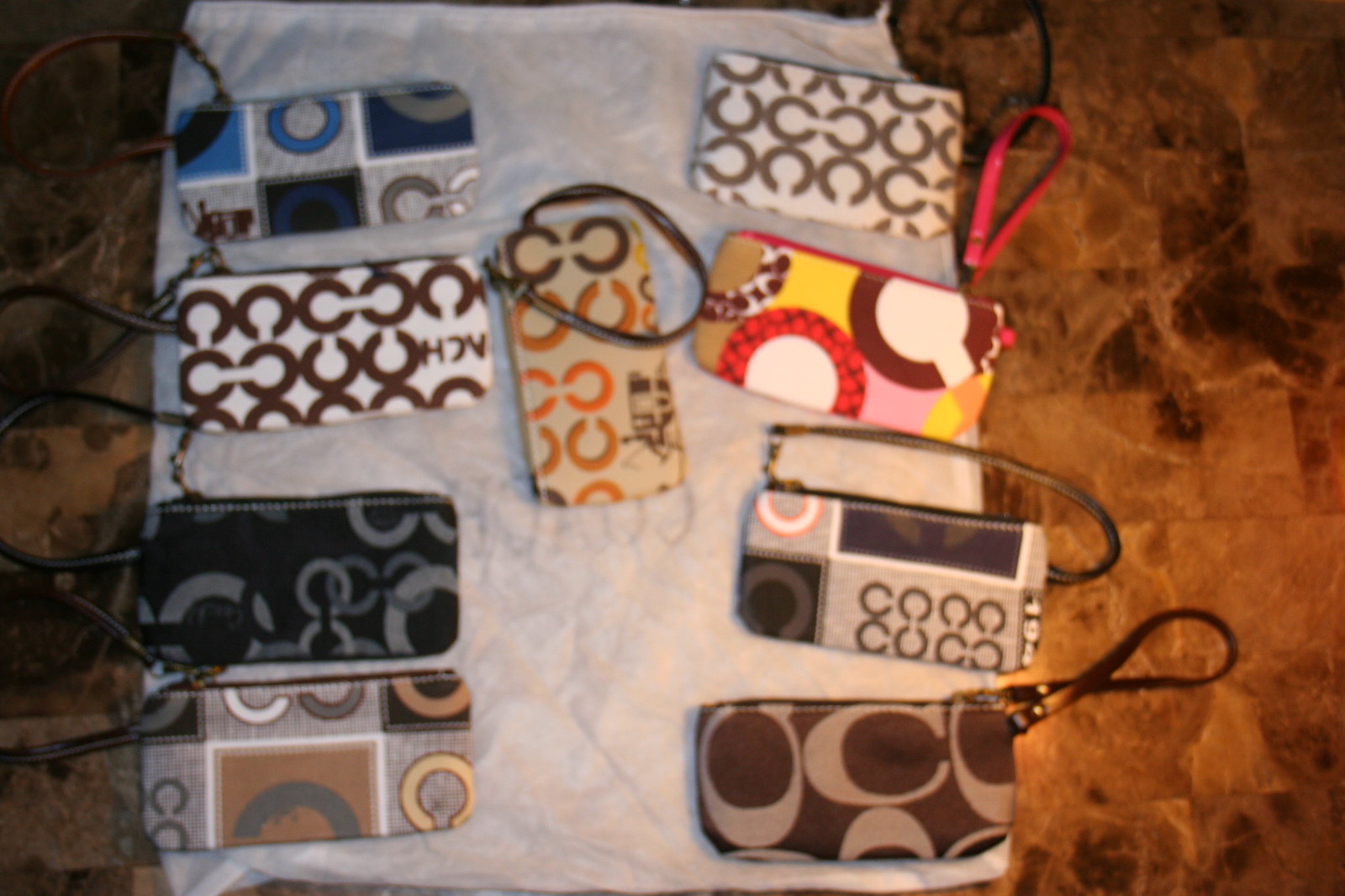This image depicts nine coin purses, each adorned with a variety of colorful patterns and circular logos, likely from high-end brands such as Coach or Chanel, with the 'C' symbols prominent on each bag. The bags are arranged with four on each side and one centrally placed, all resting on a folded white towel. The setting is either a brown tile floor or what appears to be a wooden table with an unusual texture. The purses come in multiple colors, including black, white, brown, yellow, red, blue, and pink. Each purse is roughly the size of a phone and features an attachable strap. The photo itself is dark, blurred, and poorly cropped, showing only a close-up view with little additional context, which somewhat diminishes the overall clarity and quality of the image.